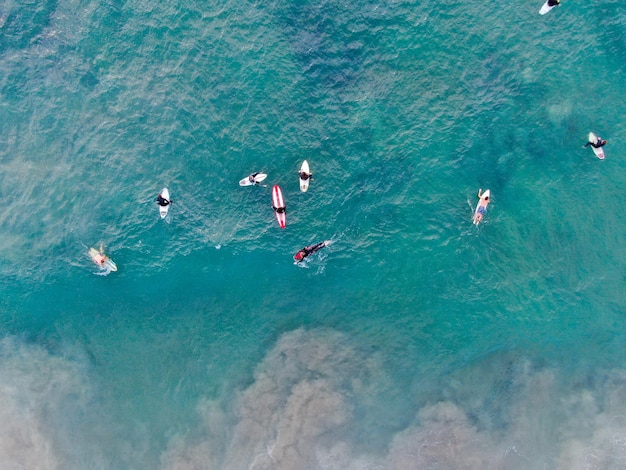A rectangular aerial photograph captures a serene, teal-colored ocean with nine tiny surfers on distinctively colored surfboards scattered throughout. The water is incredibly clear, revealing what resembles a smoky-textured coral reef beneath the surface. The surfboards are mostly white, with one sporting a blue stripe and another bearing two white stripes on a striking red background. Some surfers lay on their stomachs, paddling, while others sit with legs dangling leisurely. The image's bottom part appears almost cloud-like, where sand and dirt have possibly been stirred up, adding a surreal touch to the scene.